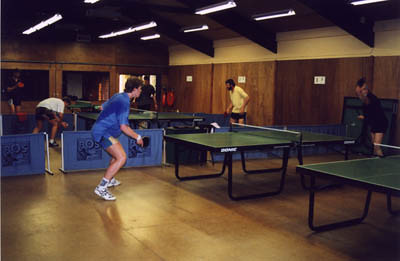In this photograph, a large, brightly lit hall is bustling with action, resembling a gymnasium or sporting event venue. The room features dark wood paneling on the walls and large wooden beams overhead, adorned with fluorescent lighting. The floor is a light tan hardwood.

In the foreground, nearest to the camera, a pair of players are engaged in a spirited game of table tennis on a green-topped table with black legs and a thin net stretched across the middle. The player on the left is a man in a blue t-shirt, blue shorts, and white high-top sneakers, visibly sweating with dark discoloration marking his shirt. His opponent across the table is dressed in black.

In the background, more tables are set up with additional pairs of players. One notable game features a player in a white shirt and dark shorts bending down for a shot, while his opponent, dressed in a yellow shirt and black pants, prepares to respond. The lively scene captures the competitive atmosphere, with at least two pairs of players engaging earnestly in their respective matches.